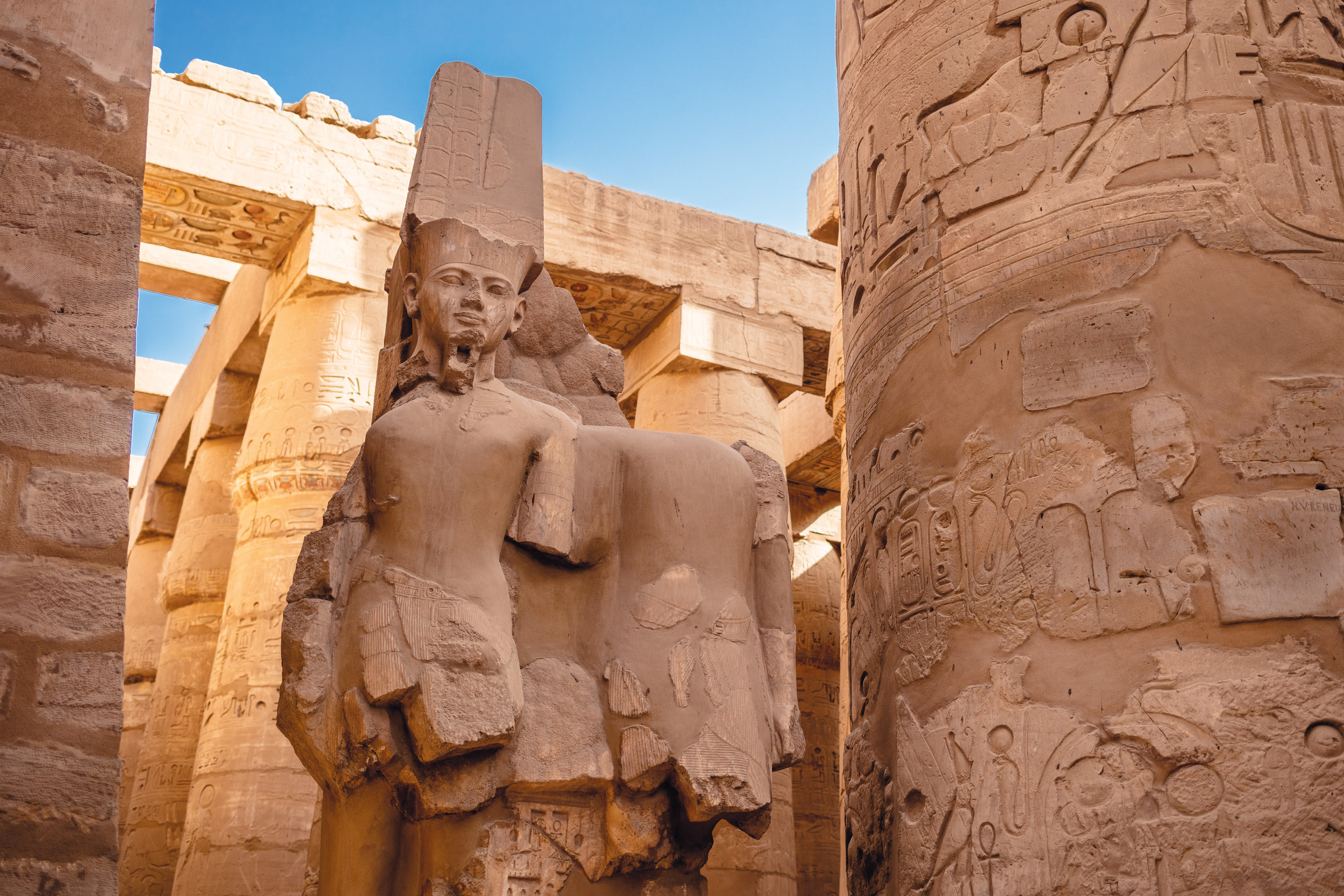The image depicts an impressive archaeological site likely located in Egypt, showcasing ancient architecture viewed from a low angle, making the structures tower imposingly over the viewer. Dominating the right-hand side of the scene is a large, rounded cylindrical pillar adorned with various intricate hieroglyphics and carvings, all etched into light brown stone. A similar pillar stands on the left, and more can be seen receding into the background.

At the center lies an Egyptian statue, characterized by its distinctive tall headdress and a partially visible robe, although the chest area appears unusually smooth, perhaps worn down by time. Adjacent to this central figure is another statue which is notably incomplete, lacking both legs and head, adding to the scene's sense of antiquity and decay.

In the background, a Parthenon-like structure can be discerned, contrasting in a much lighter, cream color. This architectural marvel is also intricately carved with figures depicting both men and women, many of whom appear damaged, a testament to the ravages of time. The entire site paints a poignant picture of ancient grandeur now weathered and fragmented.